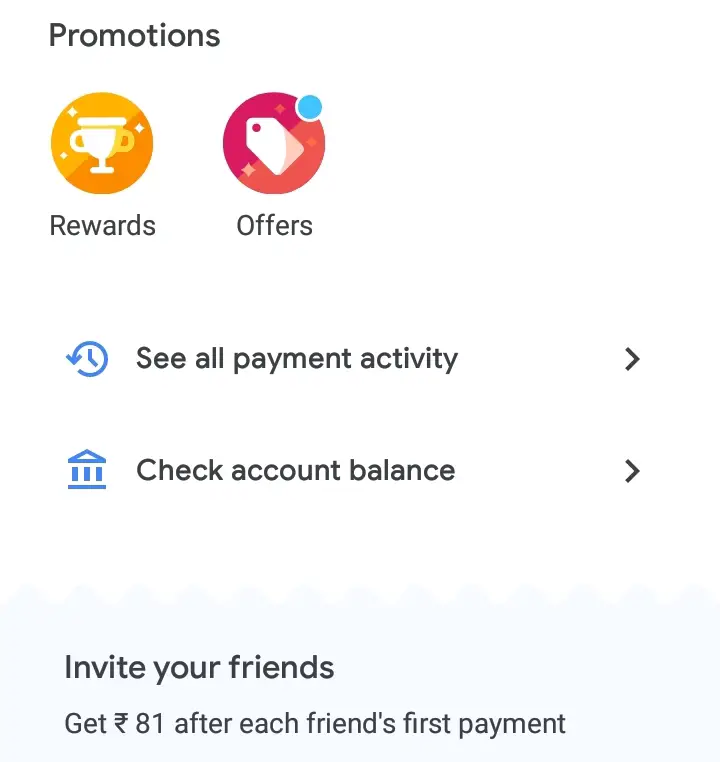This promotions page from a financial services provider features a prominent "Promotions" header in black text at the top. The page is primarily set against a white background, offering clear and bold text for easy navigation and identification. 

At the top, there are two main icons:
1. **Rewards**: Represented by a golden trophy, implying benefits or points one can earn.
2. **Offers**: This icon features a circular logo with purple and orange colors, accented by a blue indicator at the top.

Below these, the page includes a section labeled "See All Payment Activity," accompanied by a blue, backwards-running clock logo. This section suggests users can review their past transactions.

Additionally, there's a clickable section for "Check Account Balance," marked by an illustration of a bank or a significant financial building, pointing to the user's account summary.

At the very bottom, the page promotes an "Invite Your Friends" program, stating "Get 81 in [specific currency] after each friend's first payment," incentivizing users to refer new customers.

The structured layout and use of color codings, such as bold text and distinctive icons, enhance user navigation and emphasize various promotional features available on the platform.